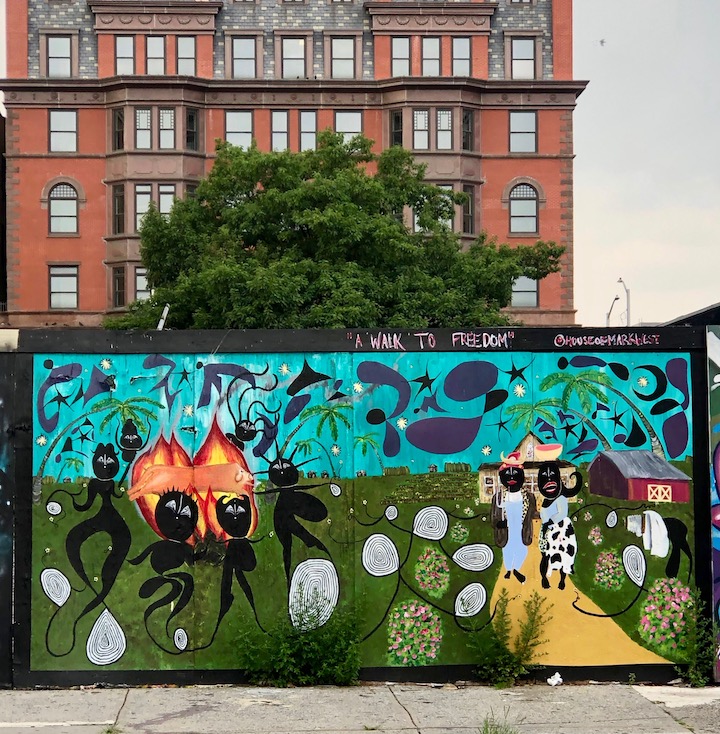The photograph captures a vibrant mural on a wall in front of a tall, multi-story apartment building with red brick walls and numerous windows, reflective of 19th-century architectural style. The building is partially obscured by the bright green leaves of a tree visible above a fence, and both the building and tree are set against a gray, cloudy sky. The mural, the main subject of the image, features a prominent black border with the white lettering "A Walk to Freedom," along with an artist's signature too small to read.

The mural itself is a complex piece of abstract art, depicting a green field under a light blue sky scattered with abstract purple shapes and stars. On the right side, a house and barn are illustrated, with two black cartoon figures walking down a path lined with bushes bearing roses. On the left, a bonfire scene shows several more abstract black figures, seemingly dancing around the fire. The figures are characterized by their simplistic, black forms with vaguely human shapes and triangle eyes, creating a somewhat eerie yet emotive atmosphere. The mural’s evocative imagery and "A Walk to Freedom" inscription suggest themes of heritage and liberation.